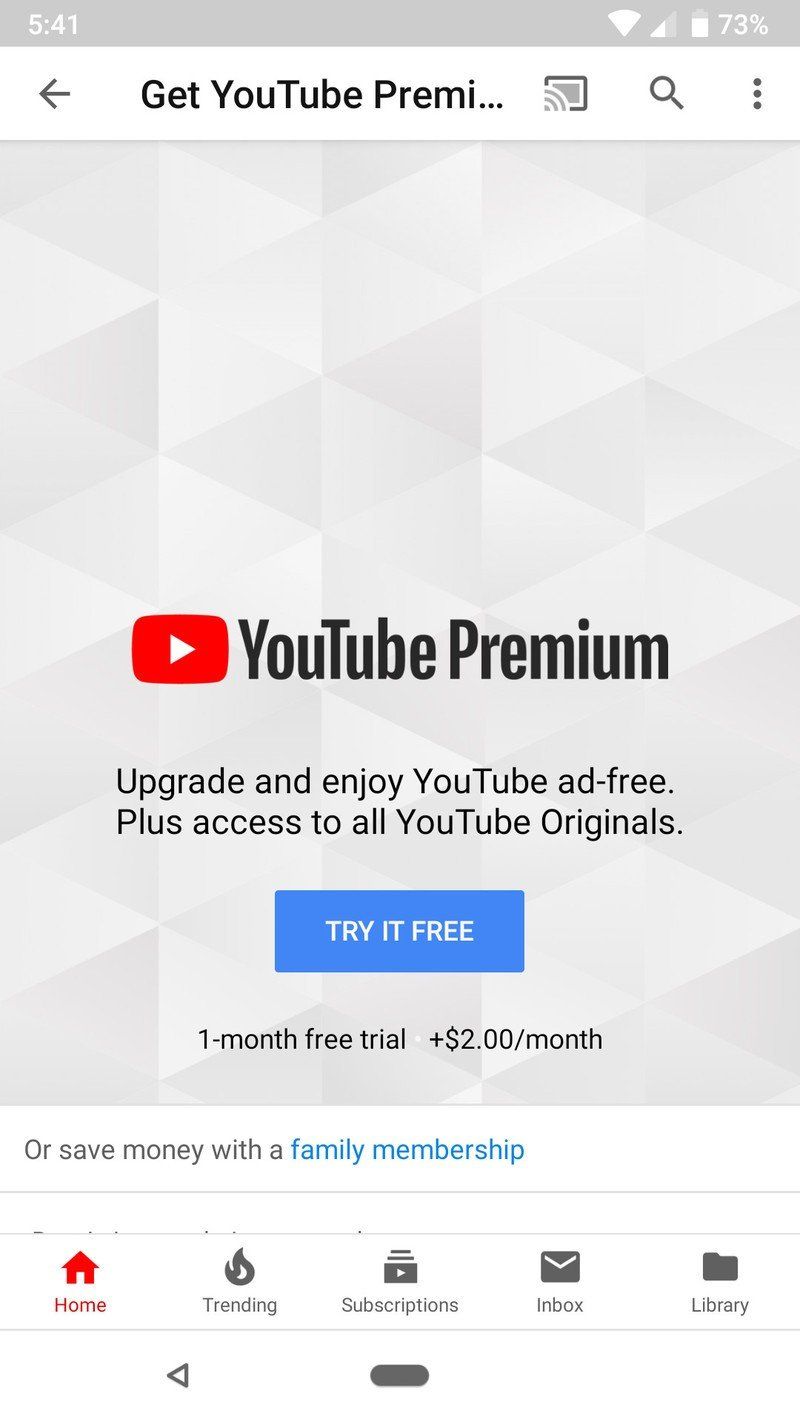This image depicts a promotional advertisement for YouTube Premium, likely appearing during the use of the YouTube platform. At the top, large black letters state, "Get YouTube Premium." Although the full word "Premium" is partially cut off, it is easily inferred. In the upper left corner, the screen displays the current time as 5:41. Adjacent to the promotional text, there is a search bar that is part of the YouTube interface.

Dominating the central portion of the image is the YouTube Premium page. This section features a prominent red square icon with a sideways triangle, traditionally indicative of a play button, though in this context, it signifies the YouTube Premium page. The heading "YouTube Premium" is prominently displayed in large black letters.

Beneath this header, the ad encourages users to "Upgrade and Enjoy YouTube Ad-Free, Plus Access to All YouTube Originals." A blue rectangular button labeled "Try it Free" serves as a call to action, enticing viewers with an offer of a free trial. Below this button, the text explains, "One Month Free Trial," and then mentions the subsequent cost of "$2 a month."

At the very bottom of the advertisement, there is an alternative offer stating, "Or save money with family membership," suggesting a cost-effective option for multiple users.